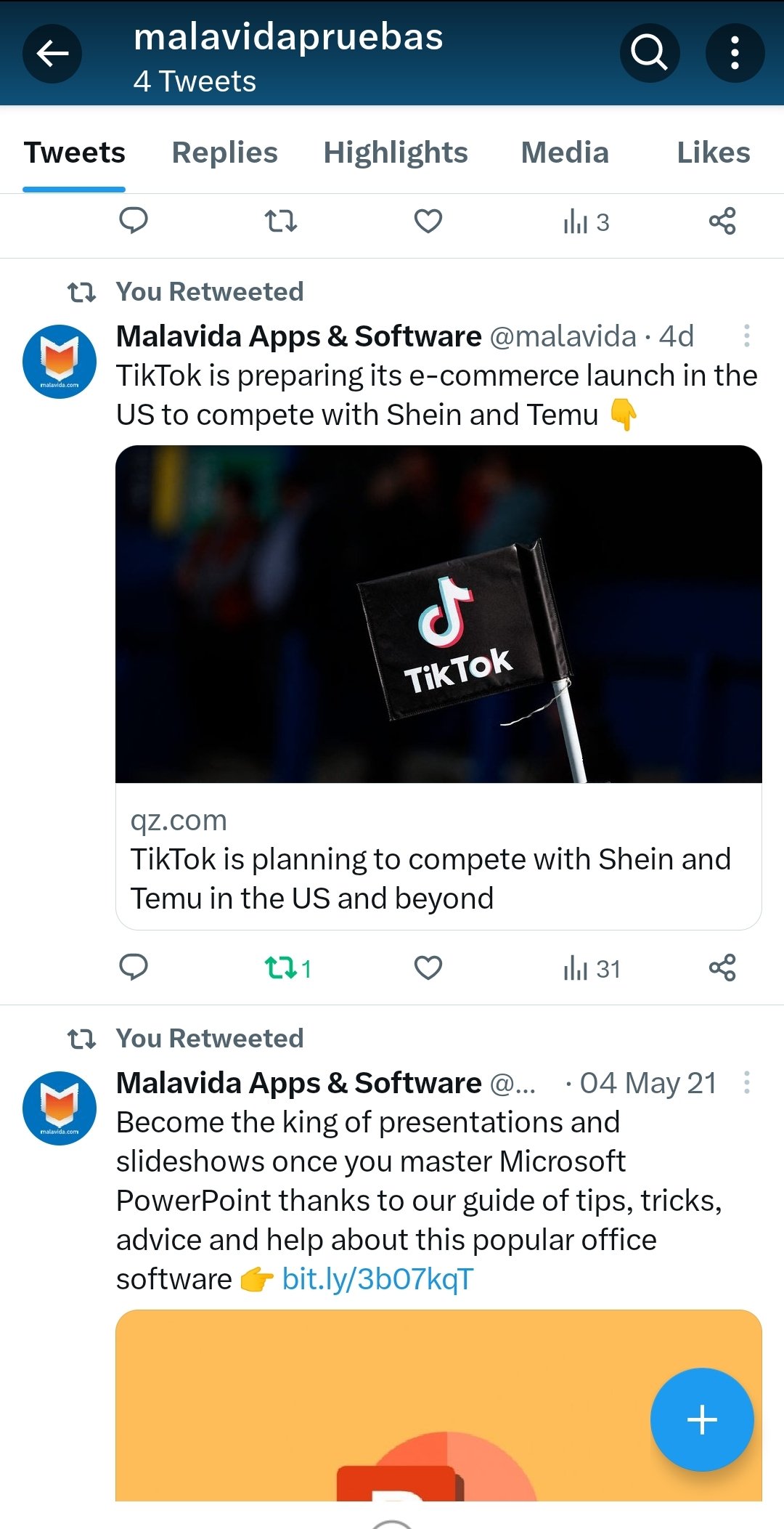This is a detailed screenshot of a Twitter profile page. At the top, there is a blue navigation bar featuring the username "Malavida Prubus" in white text. To the left of the username is a white back arrow, and to the right are three icons: a magnifying glass (search), three vertical dots (more options), and a three-line icon within dark circles.

Beneath the navigation bar, there are five tabs labeled "Tweets," "Replies," "Highlights," "Media," and "Likes." The "Tweets" tab is currently highlighted in blue. Below this section, there are five interactive icons for individual tweets: comment, retweet, like, views, and share.

Two tweets are visible in this screenshot. The first tweet shows that the user has retweeted content from "Malavida Absence Software" and "Malavida for Days." This tweet discusses TikTok's preparation to launch its e-commerce platform in the US to compete with Shein and Temu. Accompanying this tweet is an image of a flag with the TikTok logo on it.